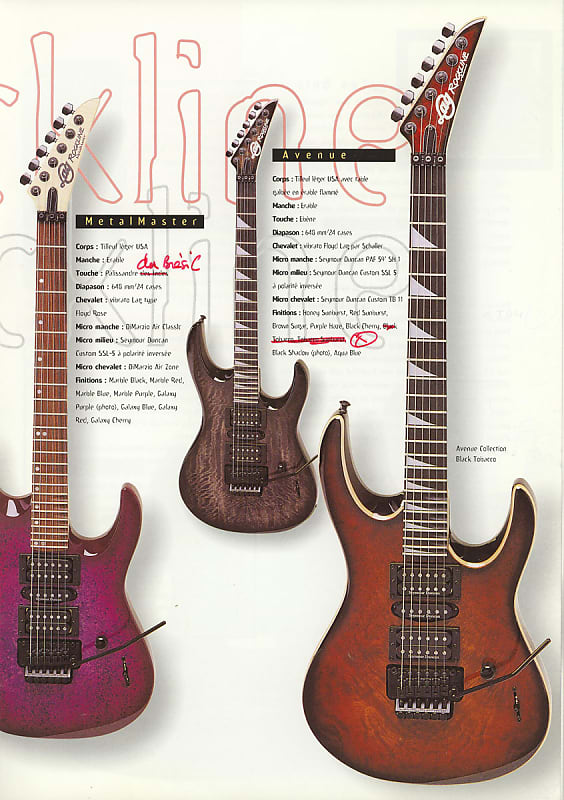The image is a detailed illustration of three different electric guitars, each prominently displaying unique designs and labels. The first guitar on the left features a magenta body with a honey-colored fretboard and a white pegboard. The second guitar in the middle showcases a dark wood grain body and fretboard with a similarly dark pegboard. The third guitar on the right has a reddish-brown body with a dark wood grain fretboard and a red pegboard area. All three guitars are of the same shape, with the left side (their right) being taller than the right side, and the bottom rounded. Each guitar has six strings and an outward-facing pedal.

Accompanying text provides further descriptions: all guitars are labeled "Metal Master Avenue," with additional specific inscriptions. The magenta guitar includes notes such as "Klein" and "Red Galaxy, Micra, Chevrolet," the dark wood grain guitar is associated with "Black Tobacco," and the reddish-brown guitar features a line crossed out for one of its descriptions. The text appears to incorporate French words like "chevalier" alongside various terms like "cores" and "touché."